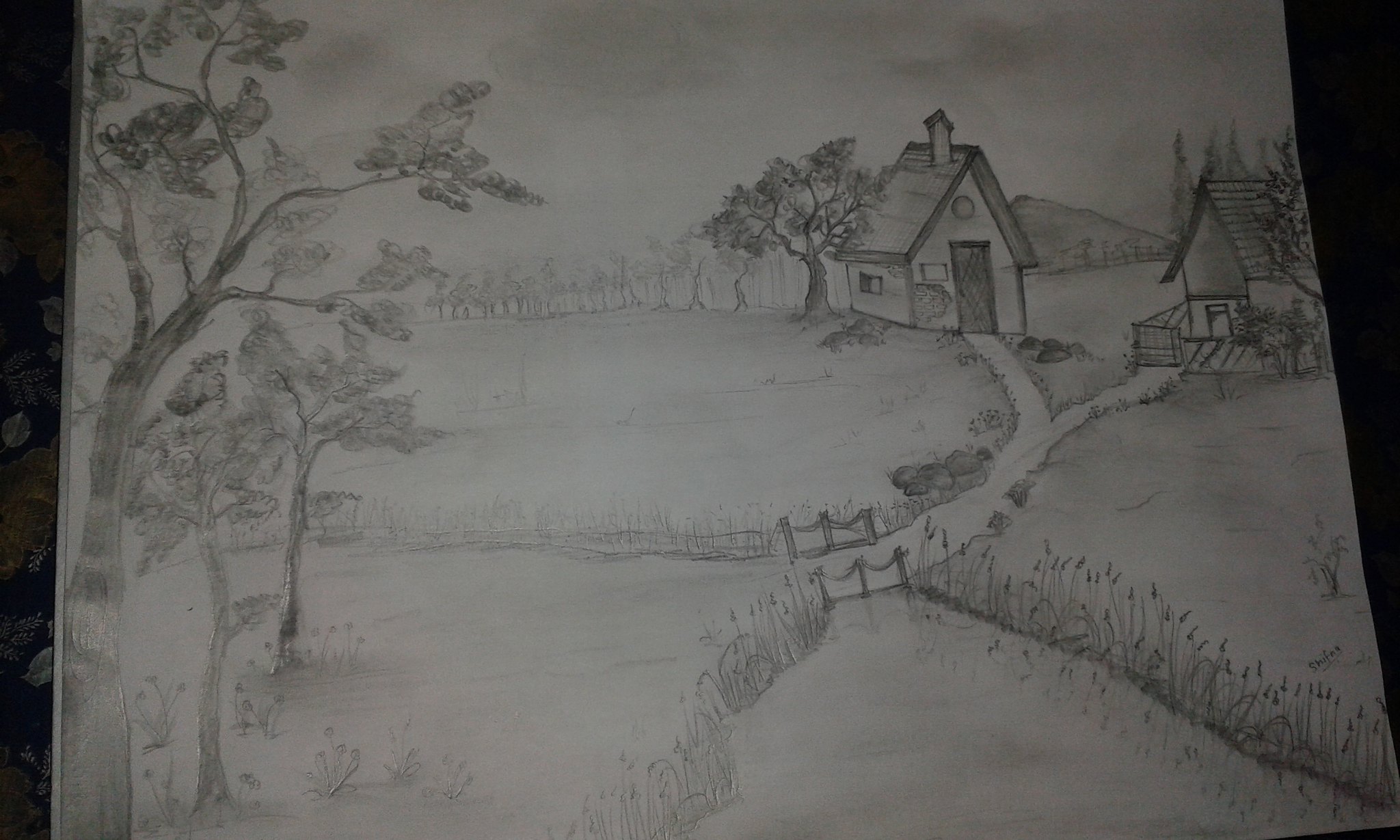This photograph captures an intricate pencil sketch on a grayish piece of paper which has been extensively shaded and detailed. The scene depicts a pastoral farm setting. On the left side, a large tree with branches and leaves towers above two smaller trees. Beneath them, small flowers add to the natural landscape. A dirt walkway winds its way from these trees, splitting off into two paths that lead to two simple houses with pointy roofs and chimneys. The house on the left, featuring a triangular roof, has a single window above a door, while the house on the right, similar in design but viewed from a side angle, has a smaller door with a path leading directly to it. In the foreground, on the right side, there is a row of flowers and a small brook with a tiny bridge connecting to the field and the houses. In the distance, a line of trees is visible, and on the upper right side, a small hill dotted with pine trees completes the peaceful, rustic scene.